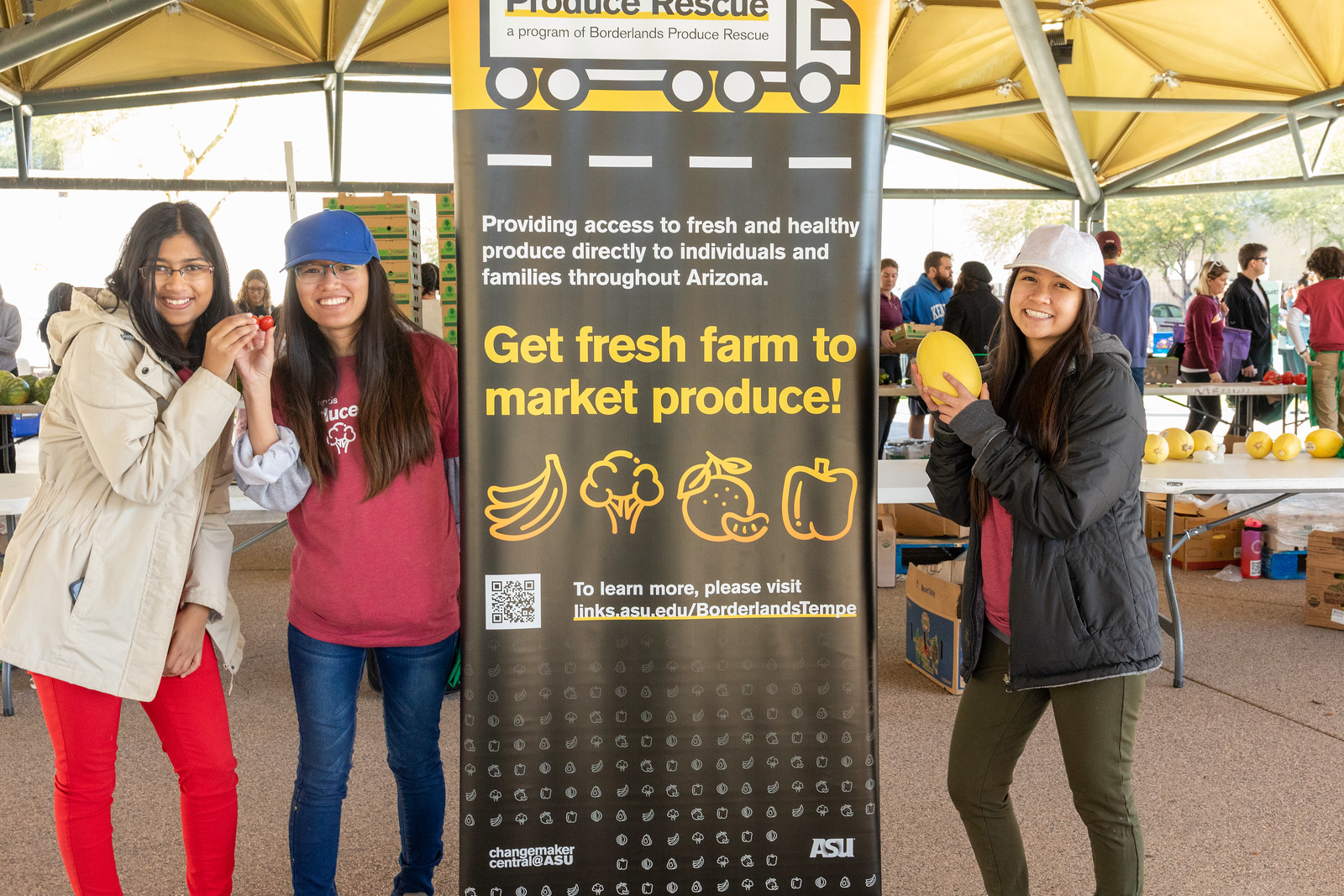In this image, three women are prominently positioned at a farmer's market, flanking a large vertical sign. The woman on the far left has glasses and long dark hair, while the one beside her, who looks similar, is also wearing a hat. On the far right, there is another woman without glasses but also donning a hat. They are standing in front of tables laden with various fruits and vegetables, with other people visible in the background, suggesting a bustling market atmosphere.

The sign in the center is detailed and colorful, with a yellow top featuring a black and white illustration of a large truck. The truck bears the text "Produce Rescue, a program of Borderlands Produce Rescue." Below this, the sign has a black background with white text that reads, "Providing access to fresh and healthy produce directly to individuals and families throughout Arizona." Further down, in yellow text, it states, "Get Farm Fresh Market Produce." There are line drawings of a bunch of bananas, a head of broccoli, an orange, and a bell pepper. At the bottom of the sign, it includes a QR code and white text that directs viewers to "links.asu.edu/BorderlandsTempe" for more information. Additionally, there is a note about "Changemaker Central at ASU" alongside the ASU logo.

The women are casually arranged around the sign, with one pair holding a small basket, possibly containing cherry tomatoes, and another holding a butternut squash, emphasizing their connection to the produce and the market environment. The photo itself has a mix of colors including black, white, yellow, tan, red, pink, and various shades of blue, lending it a vibrant, lively feel. The overall impression is of an informal, community-focused setting dedicated to promoting access to fresh and healthy produce.